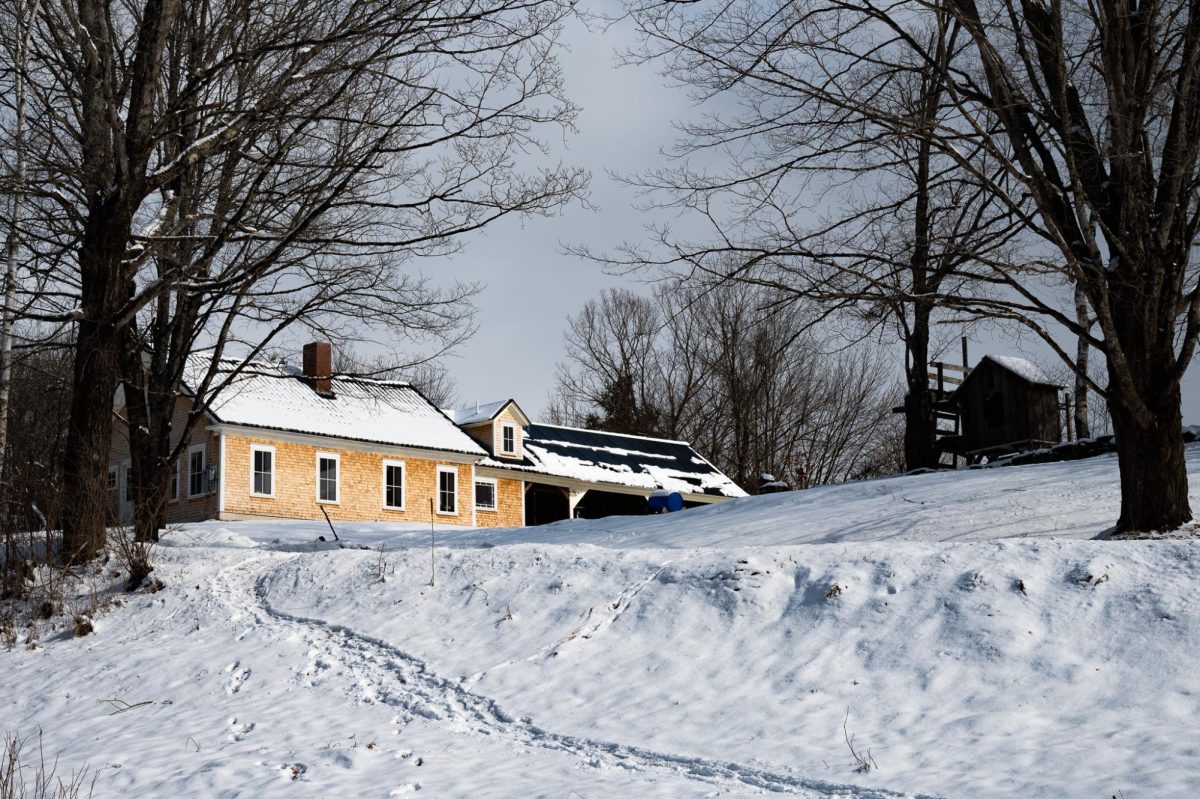The photograph captures a serene winter scene centered around a light brown stone house set against a snow-covered landscape. The house, prominently framed in the middle, features four rectangular windows with white outlines and a black shingled roof blanketed in snow, complemented by a chimney. There appears to be a covered area or garage partially obscured by a snow bank. Flanking the house are several bare trees devoid of leaves, enhancing the wintery atmosphere. In the background, a smaller structure with a triangular roof, possibly a shed or jungle gym, can be seen. Tracks in the snow, perhaps from a sled or an animal, lead towards the viewer, adding a dynamic element to the otherwise tranquil scene. To the right, atop a slight hill, there is an additional structure, a two-story building suggesting a neighboring house, completing the picturesque tableau.